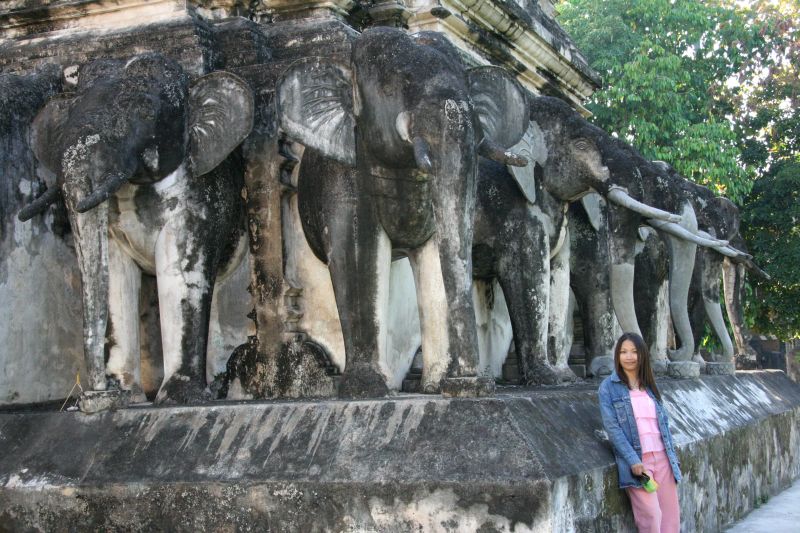In this photograph, an Asian woman with long, straight, dark brown hair, parted in the center, stands in the lower right-hand corner next to a grand statue. She is dressed in a pink tiered top, pinkish pants, and an open denim jacket. The woman holds a black and green object in her hand, possibly sunglasses, giving a hint that she may be a tourist. She is leaning against a large, weather-worn stone base that stretches up to her shoulders and is chamfered back at the top third, lending a vertical prominence to the scene.

The focal point of the statue is the impressive arrangement of six or seven tusked elephants with long trunks, facing outward in every direction. The elephants are rendered in dark hues of black and brown, mixed with white blotches, suggesting wear and exposure to the elements. They stand atop the stone platform, which matches their worn appearance. Above them, the scene extends upward to a capstone or roof, creating an elevated structure. The background reveals some green trees to the right, adding a touch of nature to the weather-worn stone. The overall ambiance of the image evokes a feeling reminiscent of a historical or cultural site, possibly in Thailand.